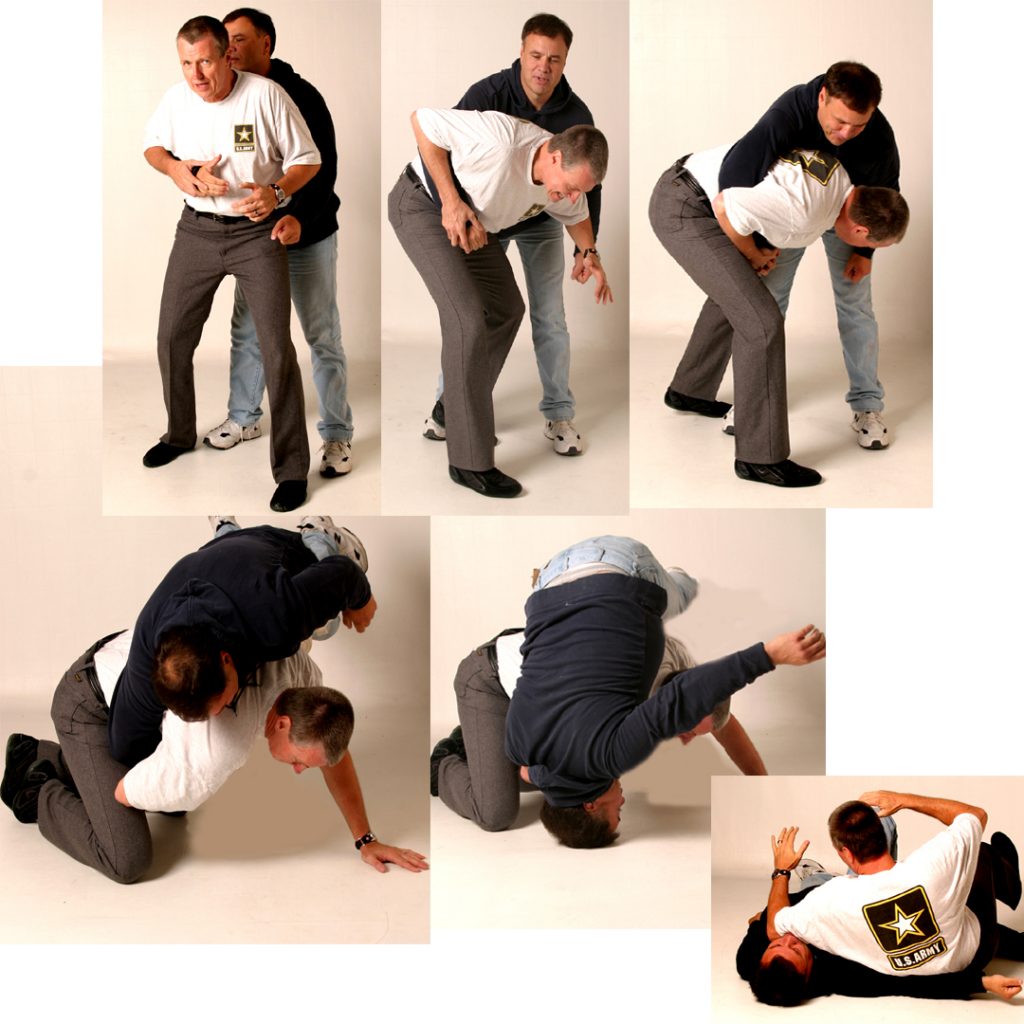The image is a composite of six sequential panels, detailing a self-defense technique demonstration. Each panel features two men; the instructor, identifiable by his white t-shirt emblazoned with "US Army" and a star symbol, and the demonstrator, dressed in a black sweater and blue jeans. In each frame, the two participants progressively perform a defensive maneuver indicating steps to counter an attacker from behind. The sequence begins with the instructor (in the white t-shirt) in front, with the man in the black sweater positioned behind him. As the sequence progresses, the instructor is shown bending forward, grabbing the attacker's arm, and flipping the attacker over his shoulder. By the final frame, the instructor has successfully thrown the attacker to the ground, pinning him down. Throughout the demonstration, the action intensifies, concluding with the attacker lying incapacitated, emphasizing the effectiveness of the self-defense technique.